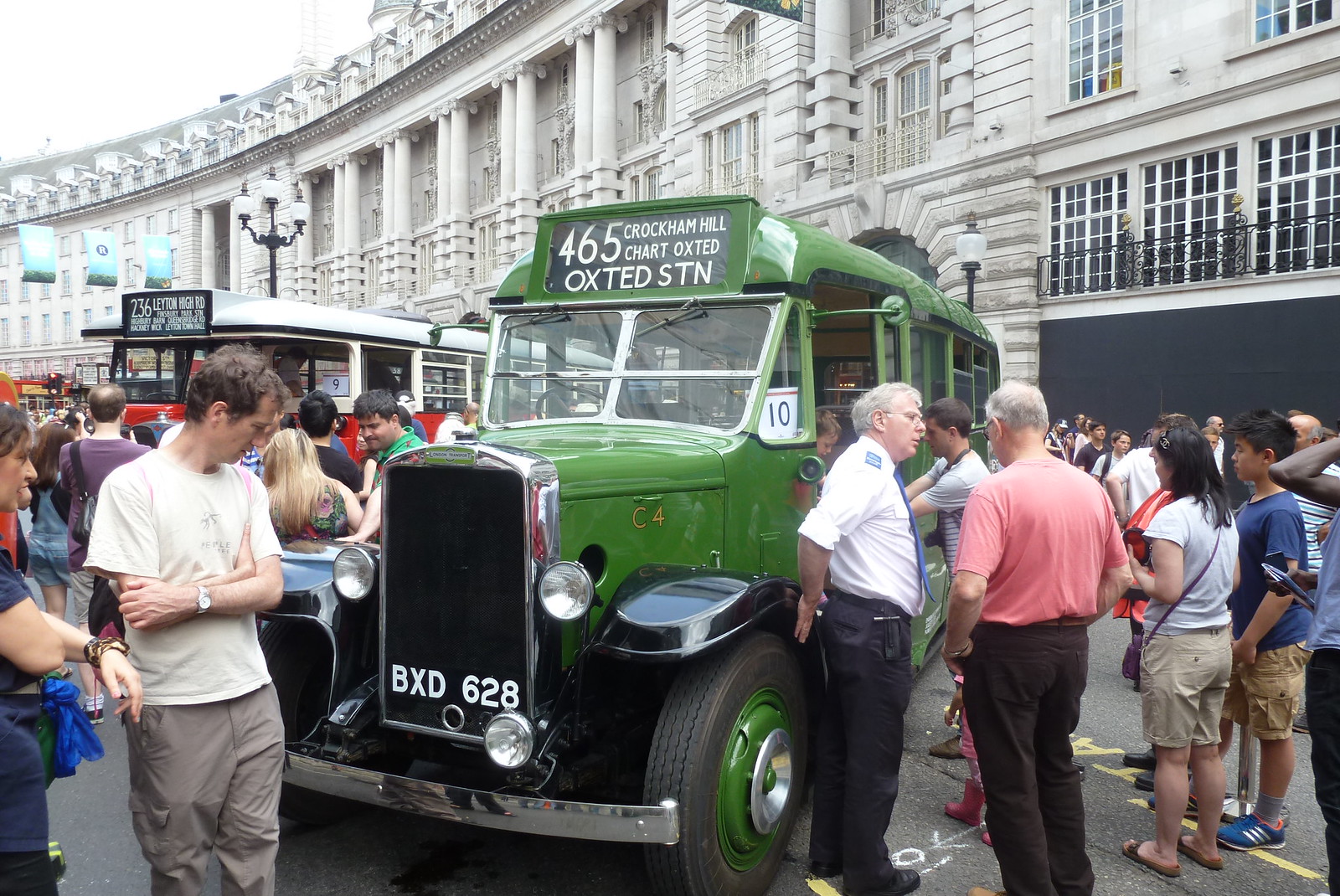The photograph captures a bustling scene centered around a vintage green shuttle bus with the number "10" displayed on the right side of its windshield. Prominently featured at the top of the bus in white lettering on a black background is the destination: "465 Cochran Hill, Chart Oxted, Oxted STN." The bus has a distinctive black rectangular grille with chrome outlines and two rounded headlights. The license plate reads "BXD 628."

To the immediate right of the bus's front wheel stands an older man in a bus driver uniform, consisting of a white shirt and blue tie. He is engaging in conversation with another person dressed in a pink shirt, brown belt, and black pants. Surrounding the green shuttle bus are numerous people dressed in a variety of colors, including a lady in blue overalls on the far left side and another in a blue shirt and black pants.

In the background, another vintage red and cream-colored bus shows the number "9" on its windshield and displays destinations in white text such as "236 Layton High Road, Finsbury Park, Hackney Wick." This secondary bus adds depth to the scene, providing a glimpse into a busy transport hub.

The backdrop of the image is dominated by a white-curved building with multiple windows and posts, trimmed in black at its top and bottom. The sky overhead appears white, and flags in blue and green hang from the building, contributing to the vibrant and dynamic atmosphere.